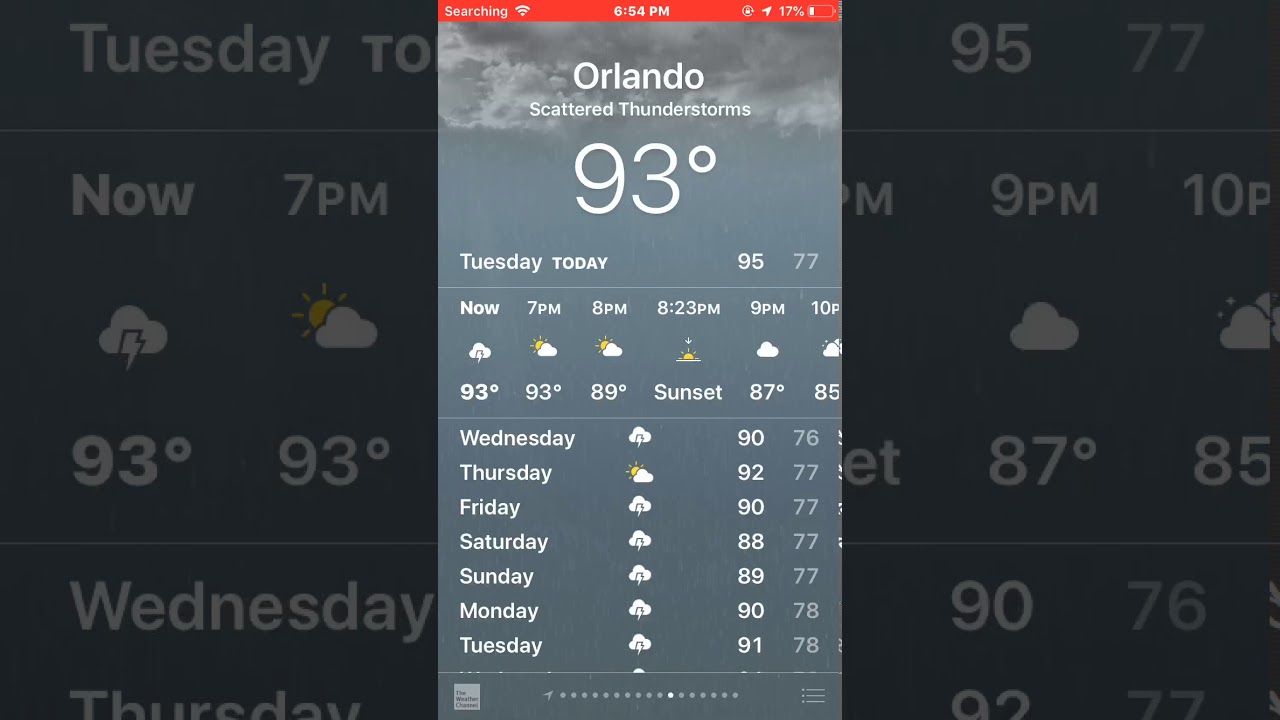The image features a smartphone displaying a weather app, with the device placed on a backdrop that amplifies the displayed data, almost resembling a presentation slide. The phone appears to be an iPhone, identifiable by the banner at the top, which includes the time centered, full Wi-Fi signal on the left, and a battery indicator showing 17% on the right, along with several notification icons.

The primary background of the app is a dark, cloudy image, which is typical of weather applications to visually represent current weather conditions. The location is set to Orlando, indicating scattered thunderstorms with a large, prominent temperature reading of 93°F in bold, white numbers. 

Beneath the main display, there is a horizontal row presenting the forecast for the upcoming hours—7 p.m., 8 p.m., sunset at 8:23 p.m., 9 p.m., and 10 p.m., showing that the rain is expected to stop after 7 p.m.

Following the hourly forecast, there is a day-by-day overview for the upcoming week from Wednesday through the next Tuesday. The forecast predominantly shows overcast conditions with temperatures varying from the 80s to low 90s, peaking at 92°F. Only one day is expected to be partly sunny, while the rest are forecasted to be overcast, reflecting typical weather patterns for Orlando during that period.